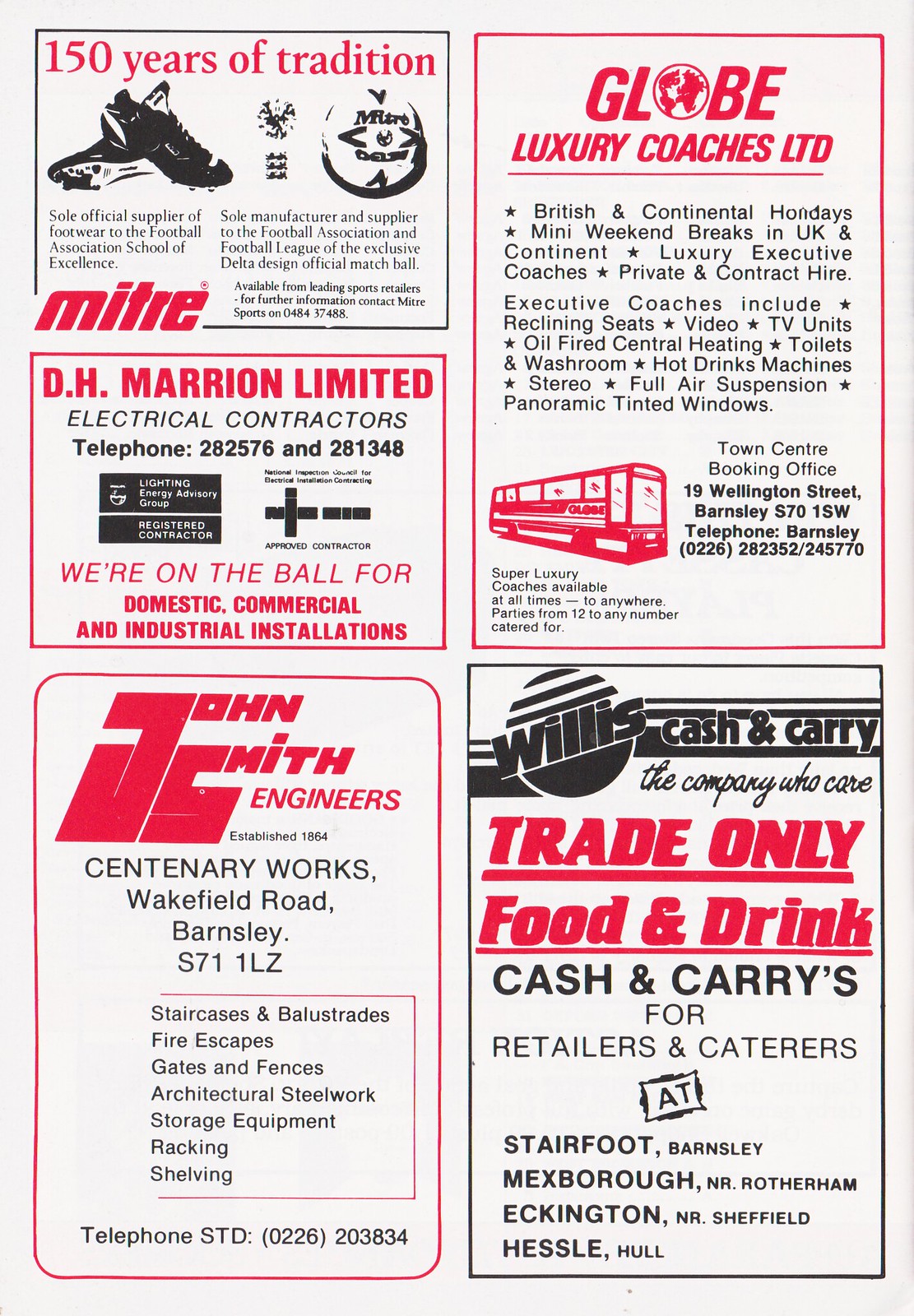A magazine page showcasing various businesses' advertisements in a traditional black, red, and white color scheme, prominently features a headline at the top left that reads "150 Years of Tradition" in bold red print on a white background. Below this, there's an ad with pictures of sneakers and a description of the manufacturer, MITRE, written in slanted red text. 

Immediately beneath this is another ad for "D.H. Marlin Limited Electrical Contractors" in red print, accompanied by their slogan, "We're on the ball for domestic, commercial, and industrial installations," and listing their contact numbers 282576 and 281348. 

In the lower left corner, "John Smith Engineers, established 1864, Century Works, Wakefield Road, Barnsley, S71 1LZ," is highlighted. The ad, with large 'J' and 'S' letters, details their services in staircases and bolsters, fire escapes, gates and fences, architectural steel works, storage equipment, racking, and shelving. Their phone number is listed as STD 0226-203834.

On the right side, an ad for "Globe Luxury Coaches Ltd" features an image of a red bus. It promotes British and Continental holidays, weekend breaks, and luxury executive coaches equipped with reclining seats, video/TV units, oil-fired central heating, toilets and washrooms, hot drink machines, stereo systems, full air suspension, and panoramic tinted windows. The address "Town Center Booking Office, 19 Wellington Street, Barnsley" and the telephone numbers 0226-282352 and 245770 are provided.

In the lower right corner, "Willis Cash and Carry" is displayed with a black globe emblem featuring 'Willis' slanted across it. The ad claims "The company who cares" in cursive, and in bold red letters, states "Trade only: food and drink." It serves retailers and caterers across various locations, including Stairfoot, Barnsley, Mexborough, Rotherham, Eckington, Sheffeld, and Hassell Hall.